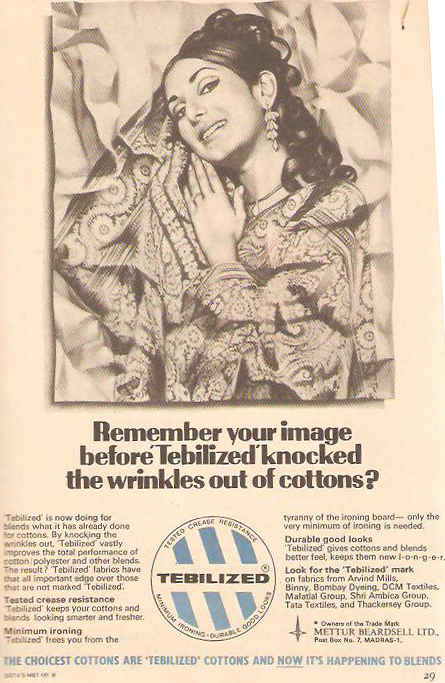The image is a full-page, colored magazine advertisement with a vintage, brownish tint, possibly from a magazine or a separate flyer. The top section features a color photograph of an Indian woman in a patterned sari, adorned with dangly chandelier-style earrings and a wedding ring on her left hand. Her thick, brunette hair is styled in a ponytail, cascading down in ringlets. She has arched eyebrows and wears heavy eye makeup, giving her a radiant look as she smiles at the camera with her head tilted slightly and one hand near her neck.

Below her image, the ad's headline reads: "Remember your image before Tabilized knocked the wrinkles out of cottons?" The text explains how Tabilized is enhancing the quality of cotton and polyester blends, reducing wrinkles, and improving fabric performance. Tabilized fabric is marketed with greater durability and a longer-lasting new look. Featured brands using this process include Arvind Mills, Bombay Dyeing, and DCM Textiles.

At the bottom, a circular Tabilized logo with blue stripes is displayed, accompanied by the slogan: "The choicest cottons are Tabilized cottons, and now it's happening to blends." The advert emphasizes that Tabilized-treated fabrics have a significant competitive edge, underscoring the importance of the Tabilized mark on textiles.